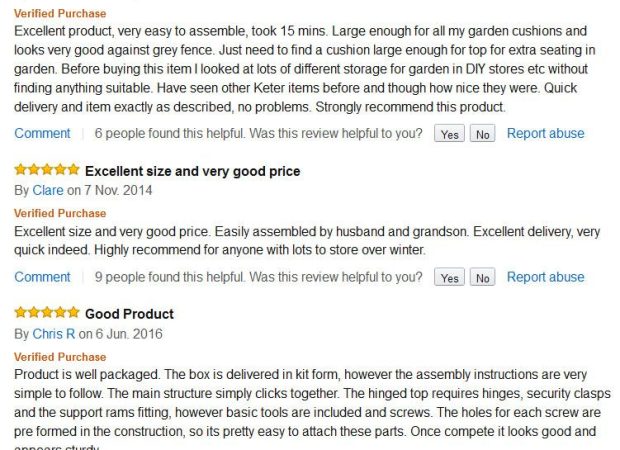**Review Compilation from Amazon: Detailed and Descriptive**

---

**Review by Anonymous on November 7, 2014**
*Verified Purchase*

*Rating: 🌟🌟🌟🌟🌟*

At the top of the review, a burnt orange label indicates "Verified Purchase." The text that follows reads in black on a white background: "Excellent product, very easy to assemble, took 15 minutes. Large enough for all my garden cushions and looks very good against a grey fence. Just need to find a cushion large enough for the top for extra seating in the garden. Before buying this item, I looked at lots of different storage options for the garden in various DIY stores without finding anything suitable. I've seen other Keta items before and thought how nice they were. Quick delivery, and the item is exactly as described—no problems. Strongly recommend this product."

Below this review, the word "comment" is in blue, followed by a note indicating that six people found this review helpful. It prompts the reader with "Was this review helpful to you?" offering options for "yes" or "no," along with the option to "report abuse."

---

**Review by Claire on November 7, 2014**
*Verified Purchase*

*Rating: 🌟🌟🌟🌟🌟*

"Excellent size and very good price," written in bold black text. Claire shares that the product was easily assembled by her husband and grandson. She praises the delivery as "excellent and very quick indeed," and highly recommends it to anyone with lots to store over the winter. Nine people found her review helpful.

---

**Review by Chris R on June 6, 2016**
*Verified Purchase*

*Rating: 🌟🌟🌟🌟🌟*

"Good product," written in bold black text, by Chris R. He explains that the product is well-packaged and delivered in kit form. The assembly instructions are simple to follow. The main structure clicks together, with the hinge top requiring hinges, security clasps, and support ramps to be fitted. Basic tools and screws are included. The pre-formed screw holes make it easy to attach these parts. Once fully assembled, the product looks good (note: Chris initially wrote "compete," corrected to "complete"). 

---

These reviews highlight the product's ease of assembly, quick delivery, and suitability for garden storage. Each reviewer strongly recommends the product, making it an excellent choice for those seeking reliable garden storage solutions.